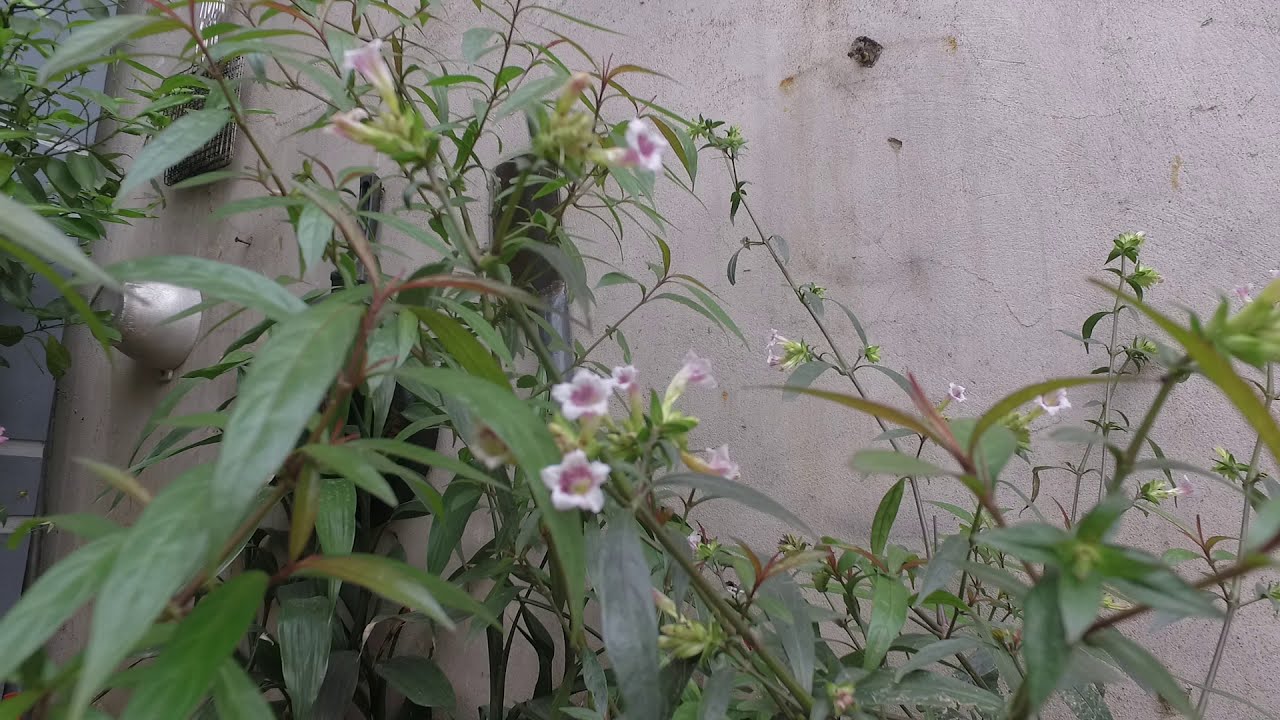The image captures a detailed close-up of a wild plant growing in front of a tannish gray concrete wall, featuring an air vent and what appears to be a meter on the left side. The focus of the photograph is on the plant's small, trumpet-like flowers that are predominantly pink with a purple rim inside. These flowers, positioned at a slight angle as if the camera is looking up from ground level, are surrounded by a lush abundance of green leaves and budding limbs. Though the flowers are comparatively small to the long, skinny leaves, they add vibrant touches of pink, purple, and green to the backdrop of gray and brown hues of the wall, creating a striking contrast. The wall likely belongs to a building, suggesting the scene is set in a garden or naturally overgrown area.